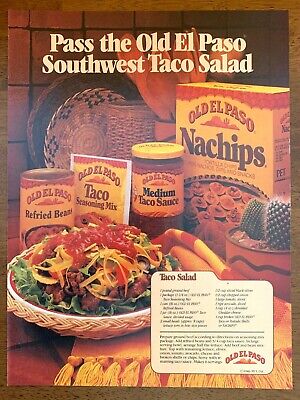The image is a vintage magazine advertisement, depicting a vibrant color photo that invites readers to "Pass the Old El Paso Southwest Taco Salad." Central to the ad is a well-made taco salad topped with lettuce, beef, cheese, and salsa. Surrounding the salad are various Old El Paso food products including a can of refried beans, a package of taco seasoning mix, a jar of medium taco sauce, and a box of nacho chips. In the background, wicker bowls and decorative tiling add to the Southwestern theme, while a small pot with two cactuses sits on the right side. A red and yellow tasseled tablecloth provides a colorful base for the display. On the bottom right corner of the ad, there's a partially visible taco salad recipe, though some of the text is blurred. The overall setup creates a warm and inviting presentation of Old El Paso’s range of products, perfect for making a Southwest taco salad.